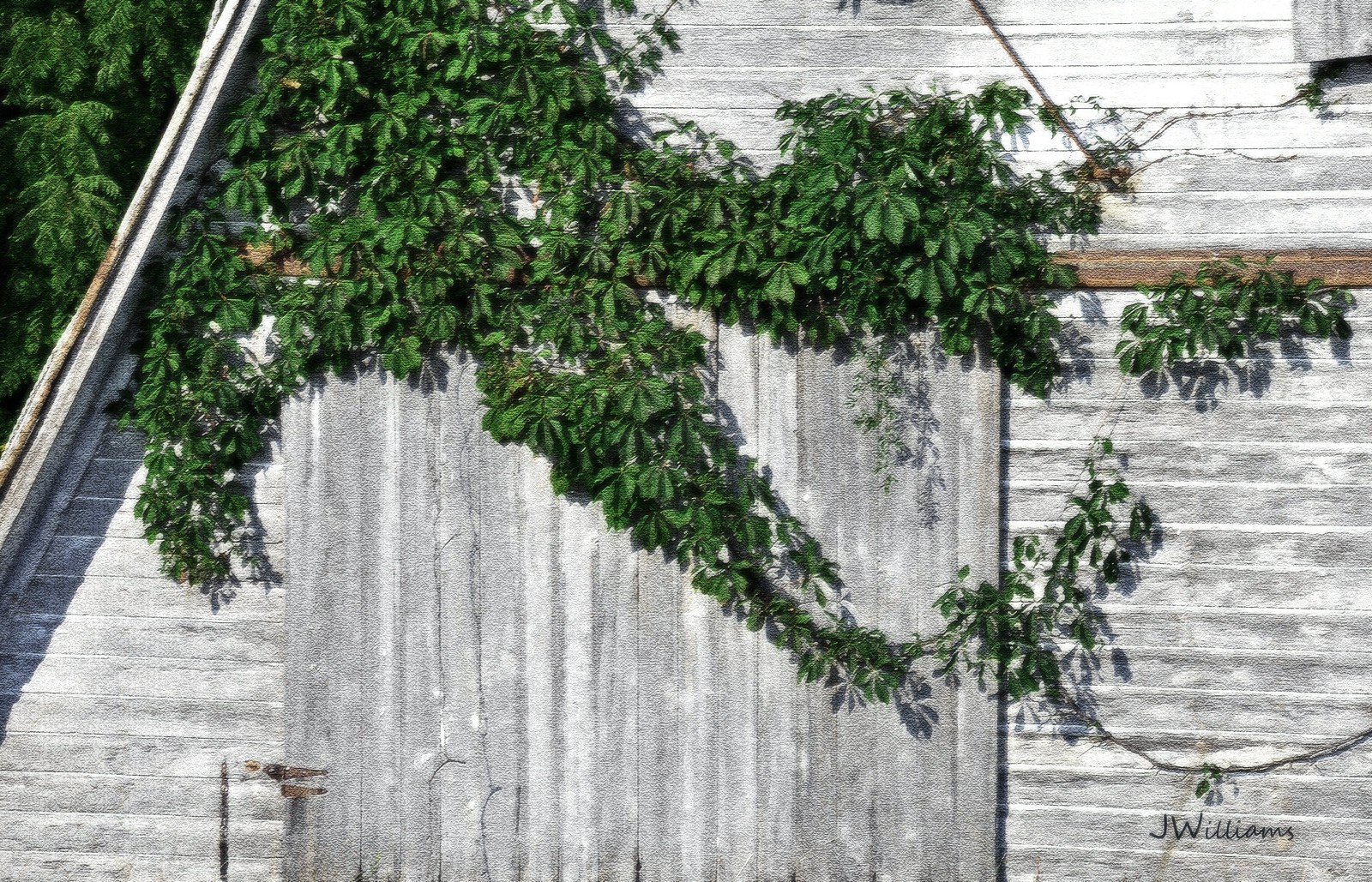The image depicts an old, weathered barn or shed with noticeable signs of age and distress. The structure features white vertical wooden slats, some of which have faded to show underlying shades of black and gray. The door is constructed with vertical boards, while the siding of the building runs horizontally. The roof appears diagonal and is adorned with an arch, over which ivy-like branches cascade down, contributing to the building's rustic charm. 

In the top left corner, a pine tree occupies much of the triangular section, while additional vine-covered trees cover approximately 40% of the building. In the bottom left, rusted hinges hint at the barn's age. A distinctive detail includes a copper-colored bar running along the base of the roof. 

On the middle right side of the facade, one of the boards stands out with a brown, painted appearance, contrasting with the rest of the structure’s penciled grayish and whitish color. 

The image, which appears to be a finely detailed pencil drawing, is signed by J. Williams in the bottom right corner—"J" in print and "Williams" in cursive. There is also an unidentifiable rectangular item in the upper right corner of the image, adding an element of intrigue to the scene.